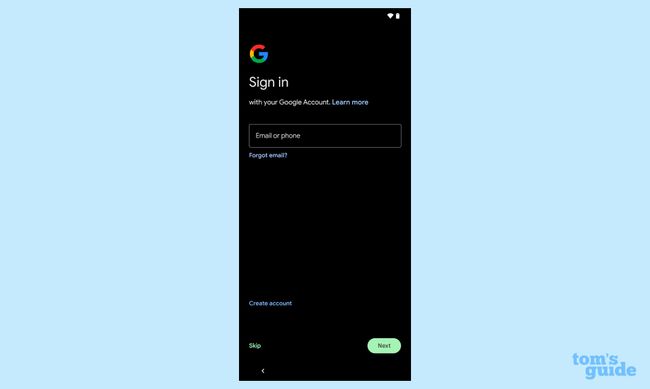The image features a blue-bordered box in the bottom-right corner with the text "Tom's Guide" in a slightly darker shade of blue. The main subject of the image is a Google sign-in screen, displayed as if on a smartphone. At the top of the screen, standard phone status icons, including Wi-Fi and battery indicators, are visible. The Google logo, a stylized "G," is prominently displayed, followed by the instruction "Sign in" in bold white letters. Beneath this, smaller white letters read "with your Google account." A hyperlink for "Learn more" is also present. 

Below these texts, a text field labeled "Email or phone" is provided for user input. Two hyperlinks are listed underneath: "Forgot email?" and "Create account," offering additional navigational options. Towards the bottom-left corner of the screen, the word "Skip" serves as another option, while on the bottom-right, there's an oval-shaped "Next" button. At the very bottom-left, an arrow icon, resembling just the tip of a traditional arrow, indicates a navigation option to go back. This detailed depiction is encompassed within the feature presentation of "Tom's Guide."